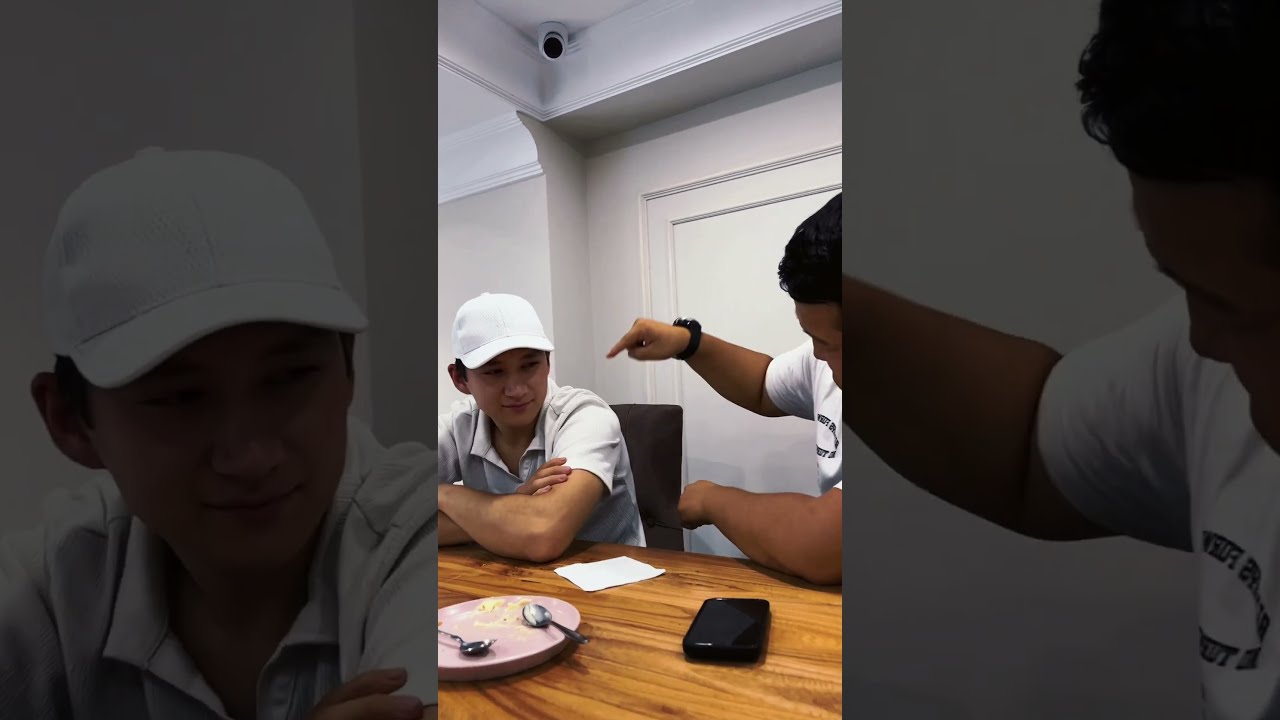The photograph captures a domestic setting, focusing on a wooden table where two men are engaged in a conversation. The man on the left, who has olive skin, wears a white baseball cap and a white polo shirt, and his arms are folded on the table. A white napkin is placed beside his left elbow. He is partially visible, with only his arms and the top part of his head and face in the frame. The man on the right, who appears slightly larger, is seated in a dark-colored, high-backed chair. He is leaning forward with his arms crossed on the table, actively gesturing towards the man in the cap with his other hand, which sports a black watch. Between them, on the wooden table, rests an empty pink plate with two spoons and some ice cream residue. Beside the plate is a black cell phone. The background features white walls and a small surveillance camera mounted in the top corner. The image was taken via a phone, evidenced by the visible border of the phone in the photograph.